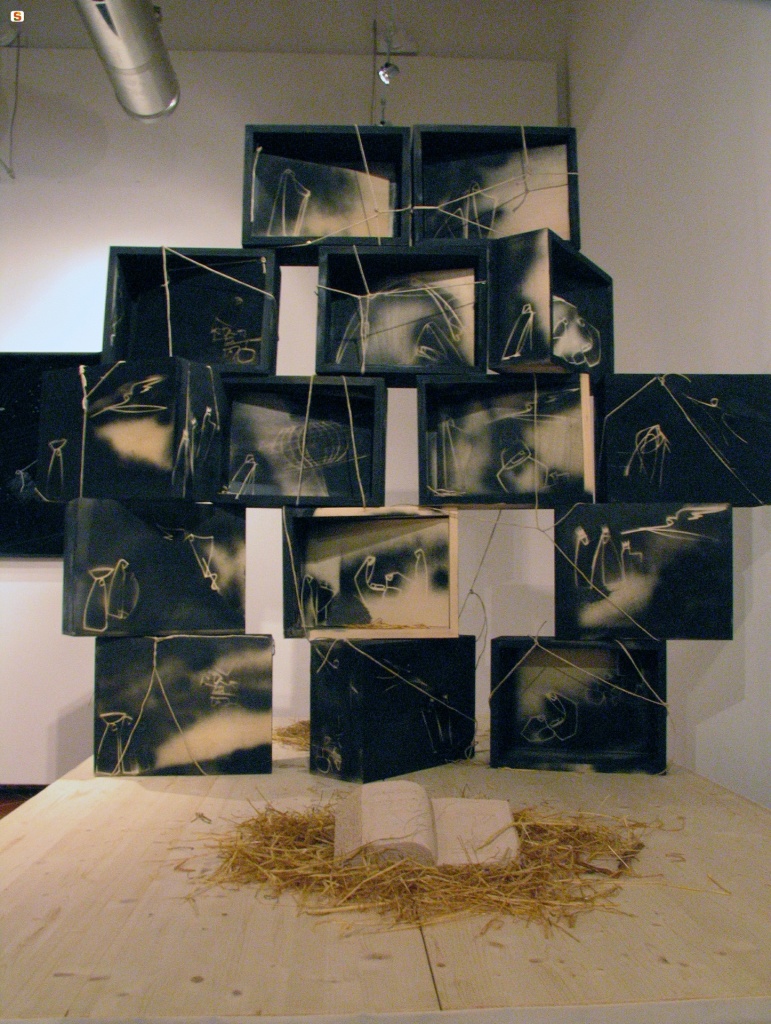This photograph, captured in portrait orientation, depicts a modern art installation within a room with light tan-colored walls. Central to the composition is a wooden platform bearing a meticulously stacked structure of dark blue and white-designed boxes. The arrangement features three boxes at the base, three on the next level, four on the third tier, three on the fourth, and finally, two boxes at the top. Notably, these boxes are not uniformly aligned; some are turned at varying angles, creating gaps between them, with only the top pair perfectly aligned and facing the viewer.

In the foreground, on the light wooden platform, there is a heap of straw cradling an open, cream-colored book or thick block resembling a book, giving an impression of an artwork. Additionally, dried wooden sticks are scattered around this central element. The upper part of the image reveals part of the room’s configuration, including the right corner and a significant detail of a metal pipe along the ceiling, hinting at an artist’s studio environment with lighting fixtures descending from it.